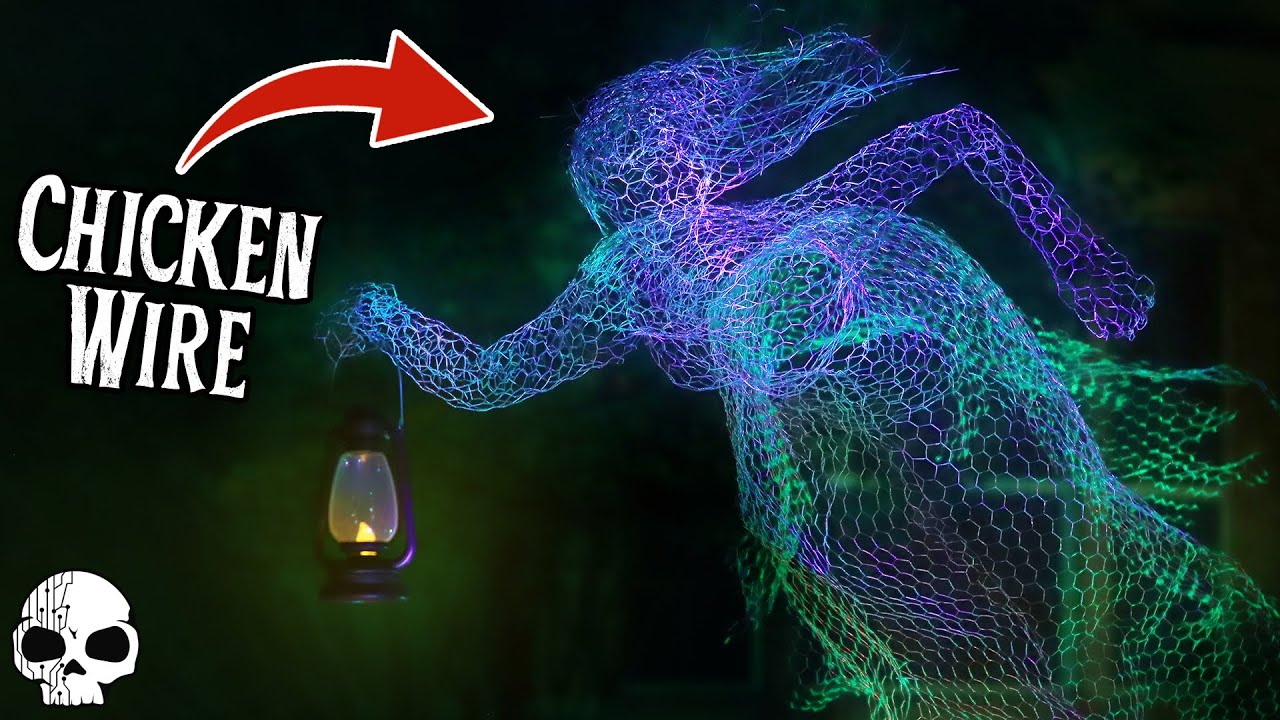The image features a striking human figure crafted from chicken wire, illuminated in vibrant shades of fluorescent blue, green, and purple, creating a neon effect. This chicken wire figure, resembling a woman with flowing hair and clad in a skirt, is depicted in a dynamic pose, bending over with her bottom thrusted up and her body lunging forward. She holds a lantern with a glass cover and a black base in her outstretched left hand. The background transitions from a dark green to a lighter green, contributing to a eerie atmosphere. In the bottom left corner, a white skull with large black eyes and visible cracks adds to the macabre feel of the scene. Additionally, white text on the left side reads "chicken wire," accompanied by a red arrow pointing right towards the figure.